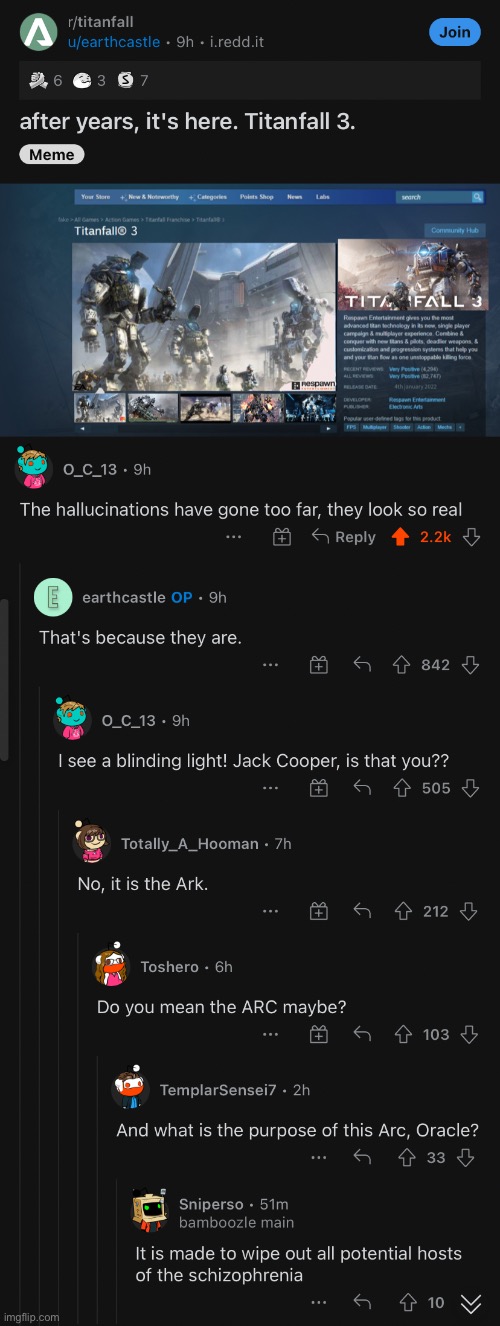This image is a screenshot of the Reddit mobile application, specifically highlighting the subreddit dedicated to the video game Titanfall. The app's interface is set against a sleek black background. 

In the top left corner, gray text indicates the subreddit name: "r/Titanfall," the standard format for Reddit community names. Beneath this, a large, bold white text exclaims, "After years, it's here, Titanfall 3," signaling the announcement of the much-anticipated game's release.

Below the text announcement, there is a prominent screenshot from the Steam website, which serves as a digital storefront for purchasing PC games. The Steam page is advertising Titanfall 3, featuring dynamic visuals that could either be screenshots, videos, or concept art related to the game.

Directly beneath the Steam advertisement, the screenshot displays user engagement in the form of comments. There are seven comments visible, each discussing or reacting to the news of Titanfall 3's release. The top comment stands out with an impressive score of 2.2k upvotes, indicating strong community approval. Each comment is accompanied by the username of the person who posted it, and options for users to reply, share, or further interact with the comments. Additional details, such as the time elapsed since the comment was posted, are also visible.

This detailed image encapsulates the excitement and community interaction surrounding the release of Titanfall 3 on Reddit, showcasing the platform's robust features for social engagement and content sharing.